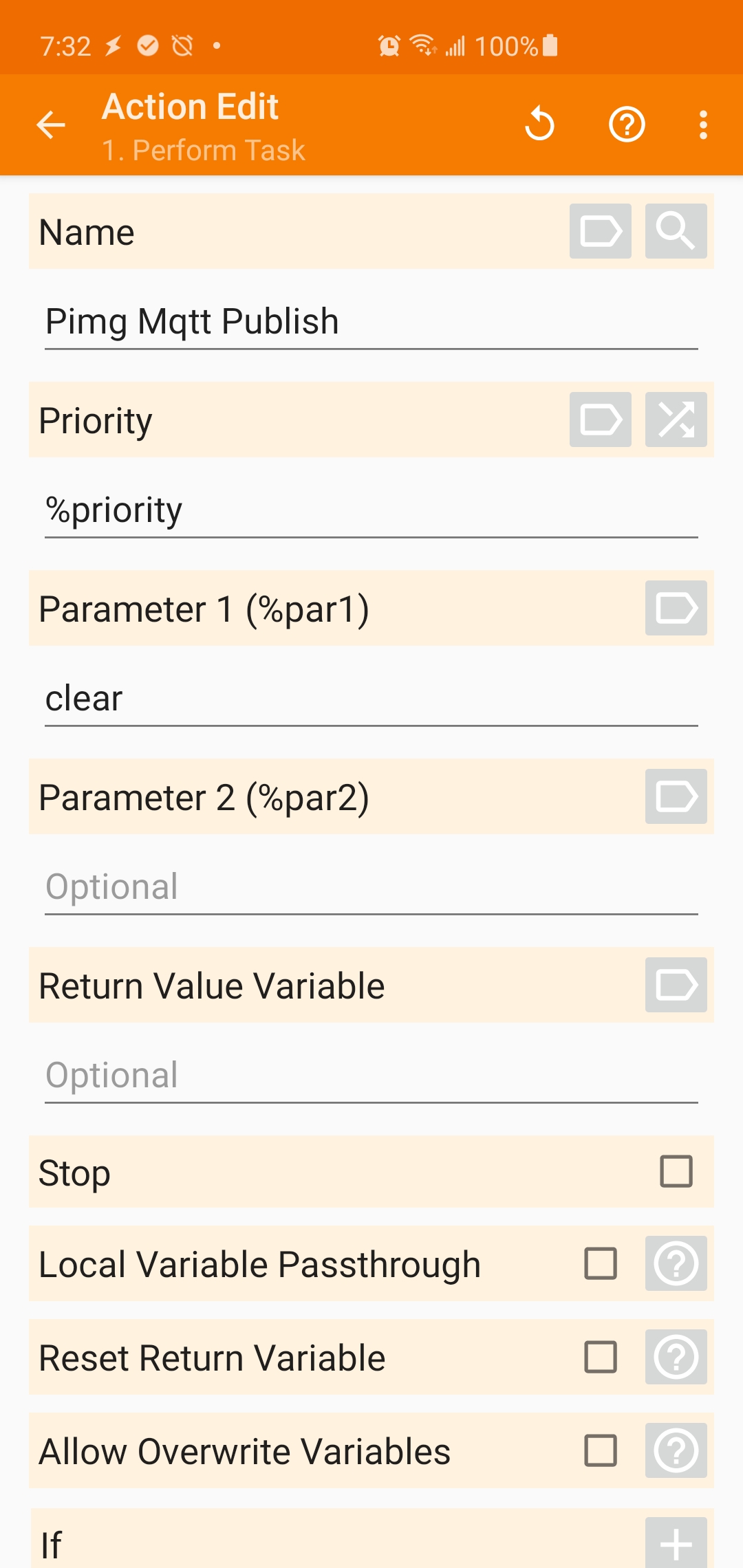The image features a predominantly white background, overlaid with various symbols and text. Central to the image is the number "732" alongside "100%", indicating a full completion or capacity. Prominently, an alarm clock icon suggests time or scheduling is involved. 

A series of action icons include:
- An edit button symbolized by a pencil,
- An action perform task indicator,
- A refresh symbol represented as two circular arrows,
- A circle with a question mark, typically representing help or additional information,
- Three vertical dots that usually imply additional settings or a menu.

The image also includes multiple instances of an icon resembling a sideways house inside a magnifying glass, perhaps depicting a search function within a specific parameter or module. 

Labels such as "P-I-M-G MQTT published priority" are present, indicating associations with MQTT protocol and prioritization. Several segments feature percentage-based priorities and parameters denoted as "Percent priority, parameter one (%P-A-R-1)" and "Percent priority, parameter two (%P-A-R-2)."

The image further details various optional return values and local variables:
- "Optional return value variable" indicated by a sideways house icon,
- "Optional stop with a square" for halting actions,
- Local variable pass-through signs represented by squares,
- "Reset return variable" also portrayed with a square and a question mark pair.

Additional configurations include options to "Allow overwrite variables" accompanied by a square and question mark, and an "if" condition bracketed by a square with a plus sign.

Overall, the image seems to focus on the detailed settings and dependencies within a task scheduling or programming interface, replete with icons representing a wide range of functions and priorities.